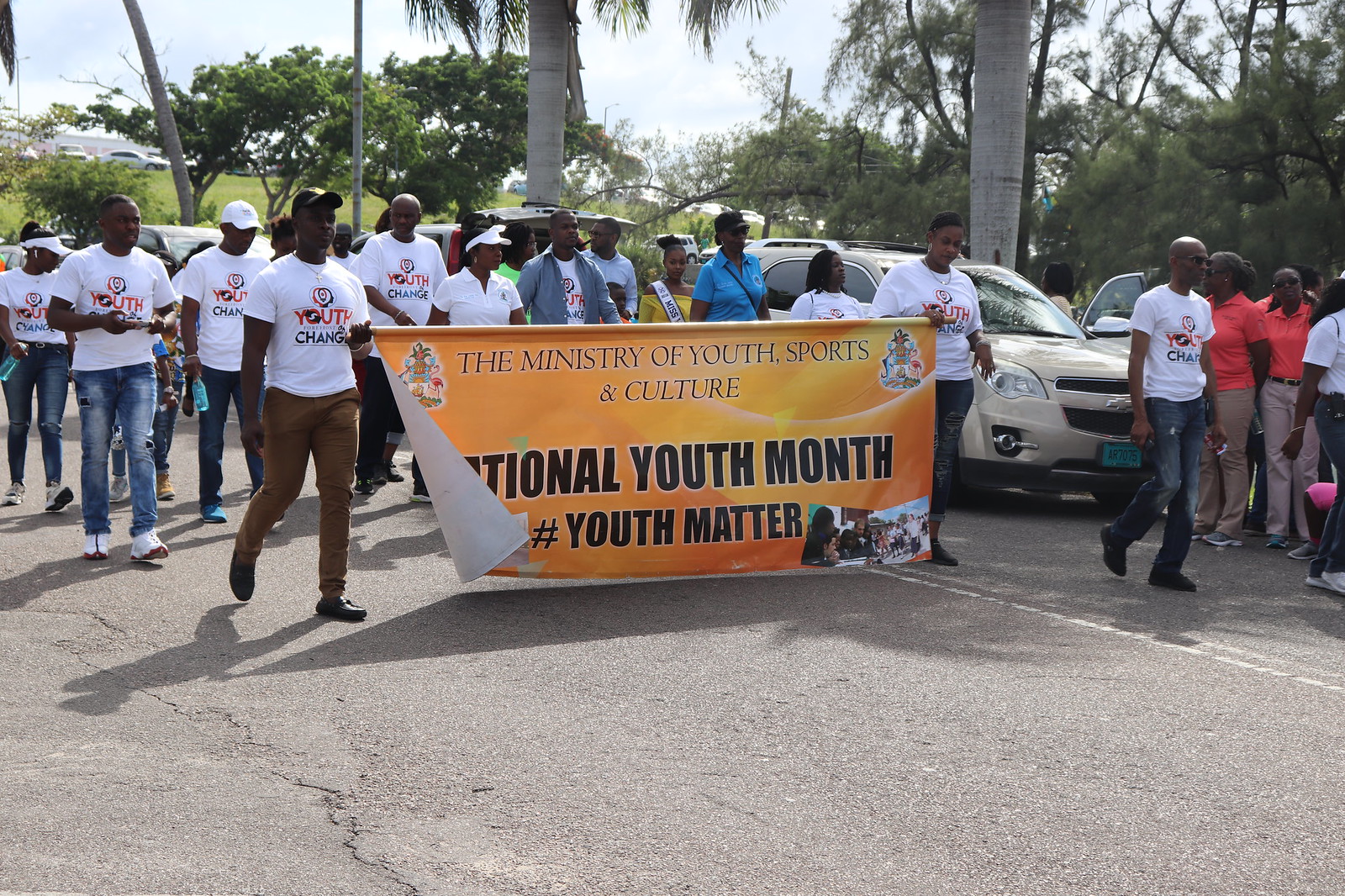The color photograph depicts a vibrant parade or march occurring on a sunlit street, framed in a landscape orientation. The central focus is on a group of dark-skinned individuals, predominantly wearing white t-shirts emblazoned with the words "Youth Change" in red and dark lettering, respectively. Leading the group are two participants holding a long, horizontally positioned banner between them on wooden poles. The banner, set against a golden background, proudly declares, "The Ministry of Youth, Sports, and Culture, National Youth Month," accompanied by crest emblems on both the left and right sides, with the hashtag #YouthMatter prominently displayed. The bottom right of the banner features images of youth, adding a personal touch. Surrounding the marchers are various spectators and additional participants in peach-colored polo shirts and red-collared shirts with chino pants, indicative of organized groups. Vehicles are parked along the right side of the street, while the scene is enriched by the natural beauty of tropical and palm trees, set against a clear blue sky. The march takes place on a street with visible cracks, adding a touch of realism to this photographic representation of the event.